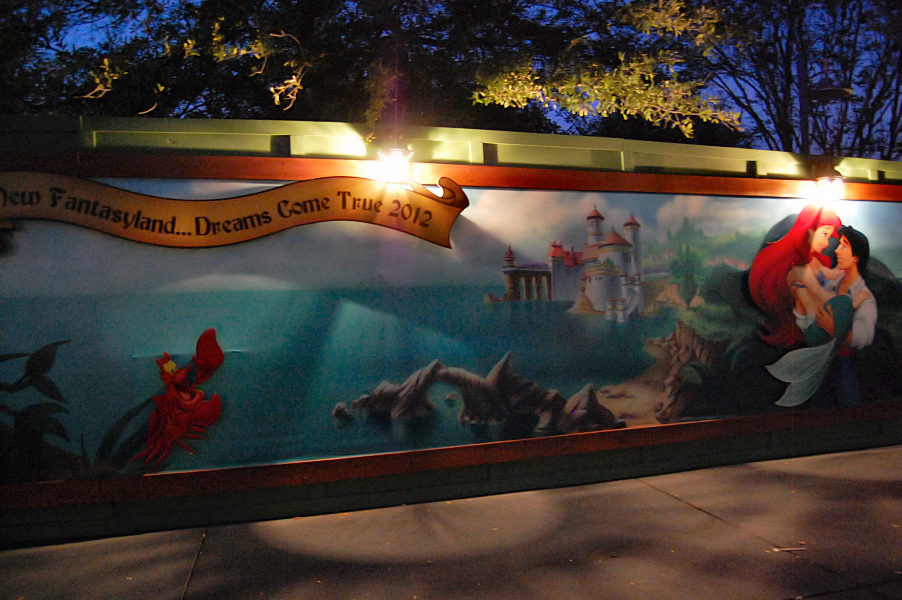This is a detailed nighttime photograph of a large mural on a construction wall at a Disney park, possibly Disneyland or Disney World. The mural celebrates "The Little Mermaid" and features prominent characters from the film. On the far right, Prince Eric is holding Ariel, the mermaid with her iconic red hair, and they gaze lovingly into each other's eyes. To their left stands a majestic white castle on the water, presumably Eric's castle, surrounded by rock formations or possibly whale fins. Further left, Sebastian the crab watches the scene unfold. Above him, a prominent scroll reads "Fantasyland... Dreams Come True 2012." The mural extends, bordered by a brown edge, with a yellow fence and trees visible above it, suggesting it's part of an ongoing construction project. The pavement below is clean, and a light illuminates part of the mural, cast against the dark night sky.